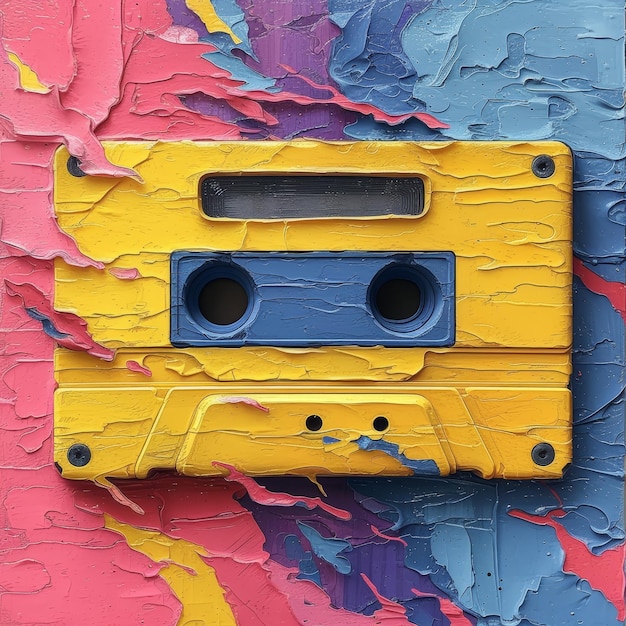This vibrant, artistic image features a striking blend of colors arranged in vertical yet loosely interpreted stripes. From left to right, it showcases a palette that transitions through medium pink, yellow, a faint strip of medium blue, medium purple, and then returns to medium blue before culminating in a gradient of lighter blue and pink. Though the stripes aren't perfectly symmetrical, they create a dynamic, visually engaging background. In contrast, the foreground highlights a cassette tape that has been whimsically painted over. The cassette's body is adorned with bold yellow paint strokes, while the areas around the wheels stand out in medium blue. The overall composition artfully juxtaposes the retro charm of the cassette tape with the contemporary flair of abstract painting.